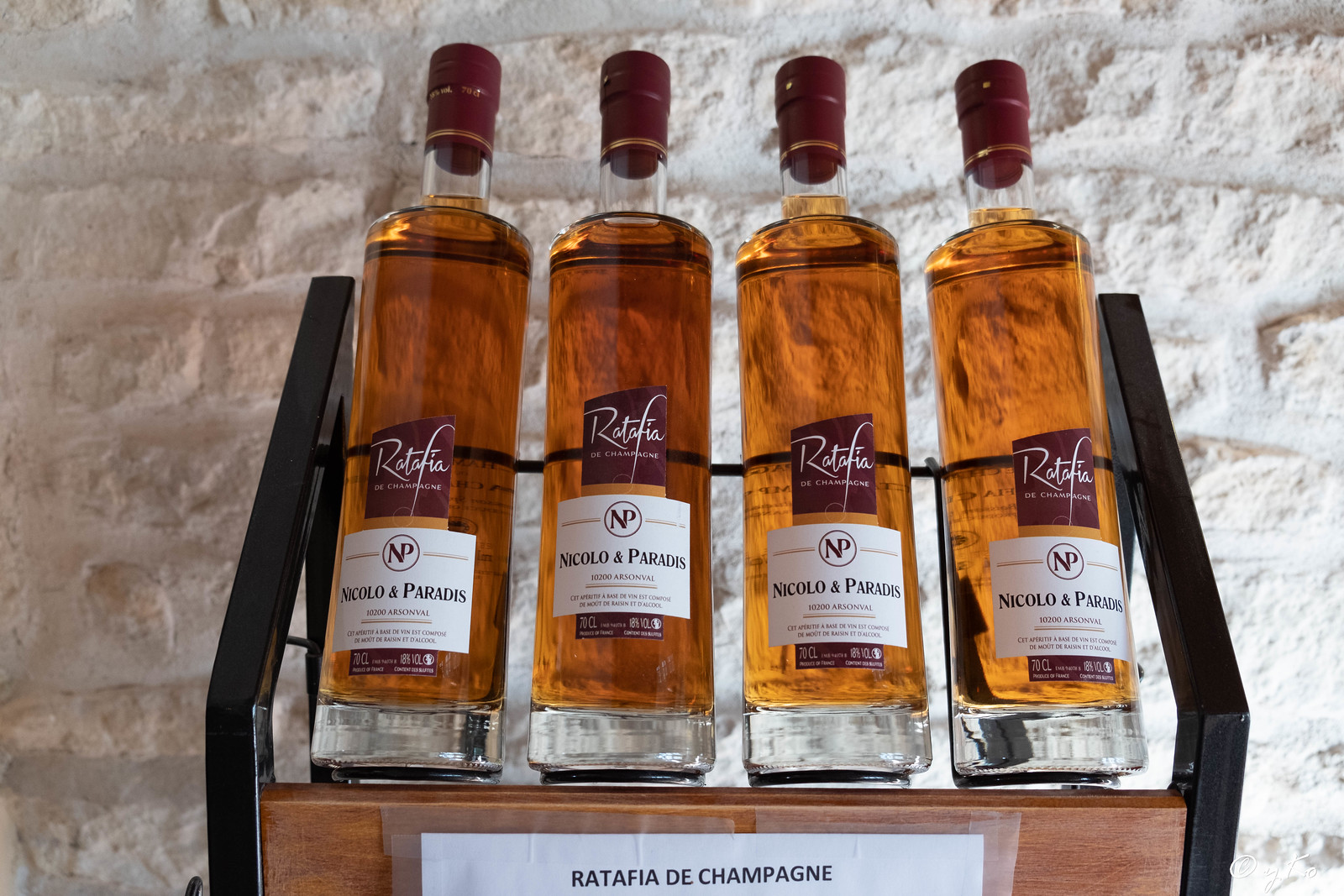The image shows a well-lit shelving unit with black handles and brown wooden platforms, standing against a white brick wall. The shelves display four glass bottles of Ratafia de Champagne, a type of foreign champagne, each with a maroon-colored cork. The champagne inside the bottles is a brownish-golden hue. A white sign is taped to the top shelf, reading "Ratafia de Champagne," indicative of the brand, Niccolo and Paradis. The bottles feature labels with a maroon background and white fonts, including details like "70 cl" and "18% volume". The white brick wall in the background, alongside the meticulous arrangement, makes the display appear sophisticated and elegant.